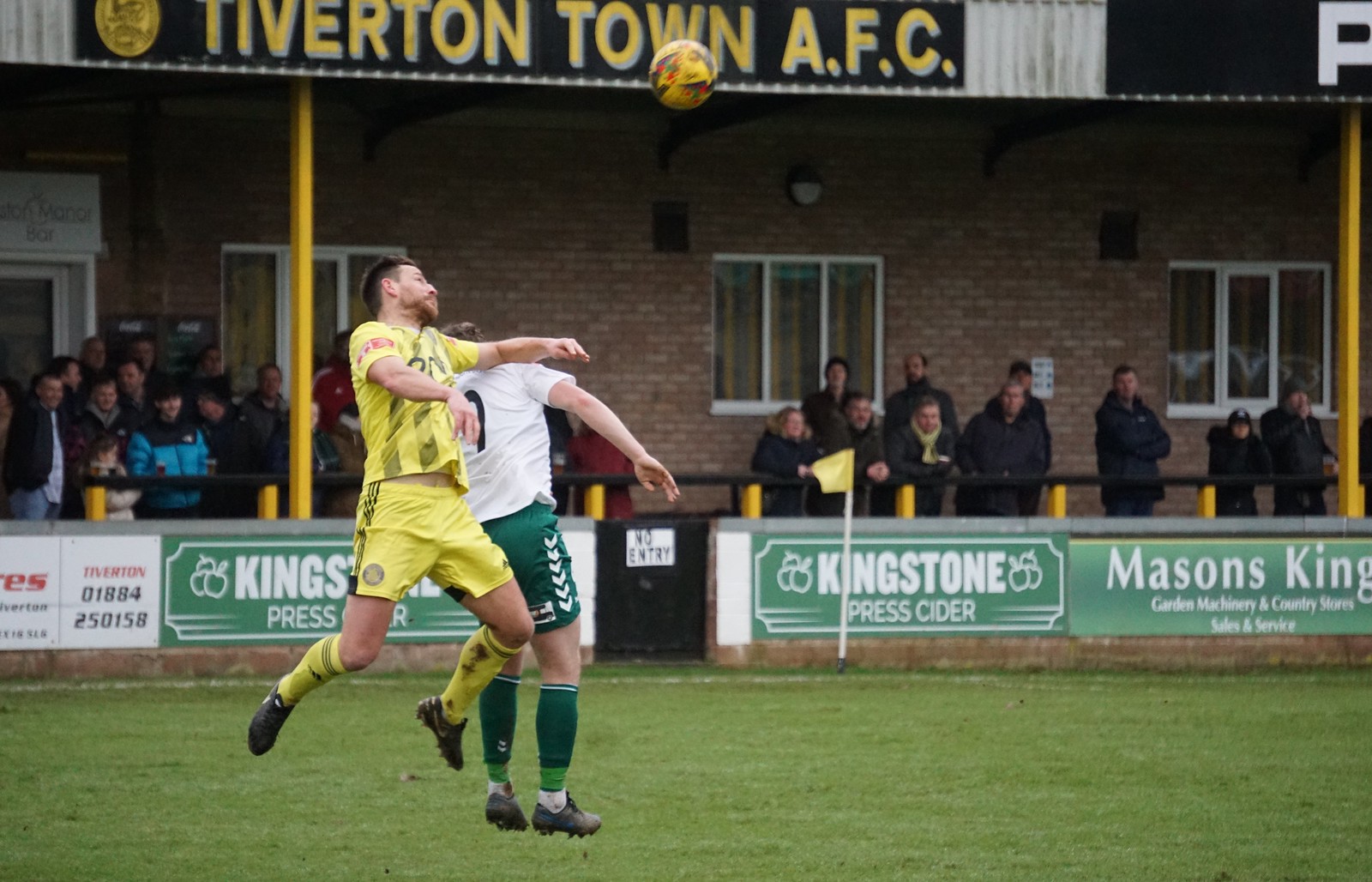On a gloomy, cold day at a soccer field, two players are engaged in an intense match on the left side of the image. The grassy pitch is green and well-maintained. The player in the foreground is wearing a yellow jersey, yellow shorts, yellow and black striped socks, and black shoes. He is mid-jump, his knees bent, and he appears to have just head-butted the soccer ball, which is captured in mid-air near the top center of the image. This player is a young Caucasian man, facing right. The opposing player, slightly behind and appearing to be losing his balance, is dressed in a green uniform with a white shirt, green shorts, green socks, and black shoes. He is also Caucasian and facing away from the camera, possibly trying to intercept the ball.

In the background, a brick building with three windows is visible. In front of the building is a brick fence adorned with green banners advertising Kingston Press Cider and Mason’s Kings, along with additional details about garden machinery and services. Above these advertisements, a black banner with yellow print states "Tiverton Town AFC," with the club's emblem to the left. Spectators, dressed in dark, wintery coats, are gathered behind the fence, intently watching the action on the field. The overall atmosphere suggests it is a chilly day, adding to the intensity and excitement of the match.